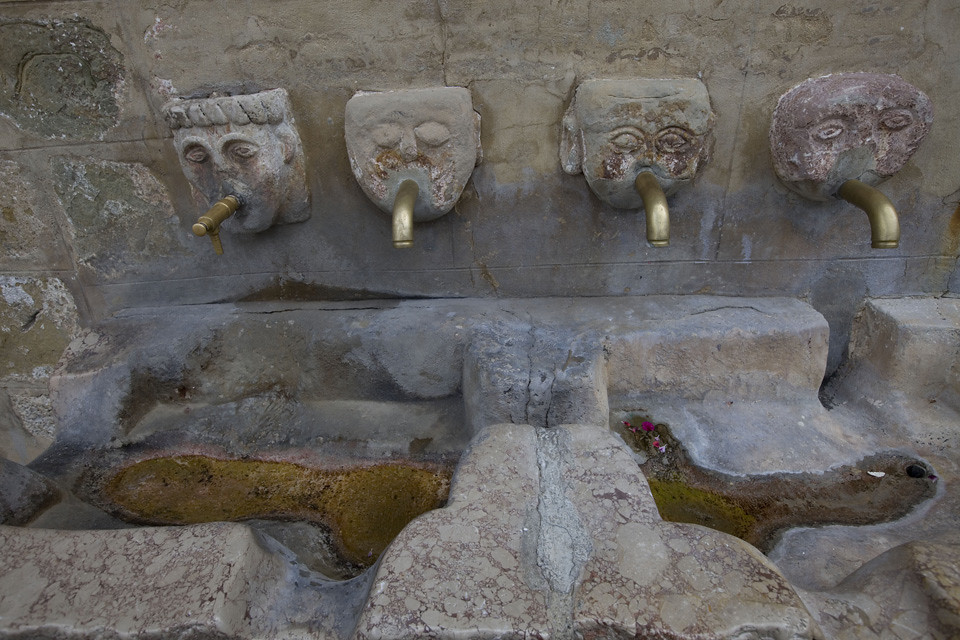The image depicts an ancient, weathered stone wall with four intricately carved faces positioned in a row. Each face, varying in detail due to significant aging, serves as the backdrop for brass or possibly gold spigots protruding from their mouths. The carvings show distinct features: the face on the far right has a flat top haircut, the next one to the left reveals just eyes and a nose, the third has large ears and pronounced eyes, while the face on the far left is badly deteriorated, only eyes barely discernible.

Each spigot extends from the mouth and curves downward, with the exception of the one on the far right, which has an additional 90-degree bend. Beneath each face, there are basins or trenches carved into the stone, likely serving as sinks or water catchment areas. The stone at the bottom shows signs of greenish moss, heightening the sense of age and exposure to elements. There are small puddles of water in two of the visible trenches, indicating recent use or residual moisture. This ancient water fixture could plausibly be part of an old bathhouse, public restroom, or communal fountain system. The entire setup is substantially worn, suggesting centuries of use.